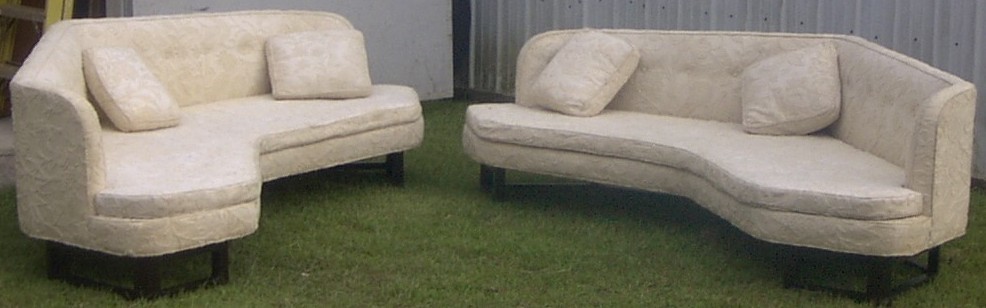This color photograph, captured in landscape orientation, showcases two uniquely designed, geometric couches positioned on a dark green surface that appears to be either grass or turf. The scene is expansive and horizontally long, emphasizing the width over height. The couches exhibit a sharp, angular, almost boomerang shape, deviating from traditional rounded designs. Each couch, spanning about 10 to 12 feet and capable of seating five to six people, is a solid light shade—white, cream, or very light gray—and comes with two matching square throw pillows. They are supported by short, black or dark brown legs, creating a subtle gap between the furniture and the ground.

In the background, the setting is framed by two distinct walls: a corrugated metal wall on the right-hand side and a plain white wall on the left. A possible window or sliding door covered with white blinds is slightly visible in the left corner, adding an element of mystery as it’s not distinctly clear. The photograph is devoid of any writing, people, animals, or mechanical objects, focusing entirely on the serene and somewhat ambiguous placement of the couches, which could be interpreted as either an indoor or outdoor setting.